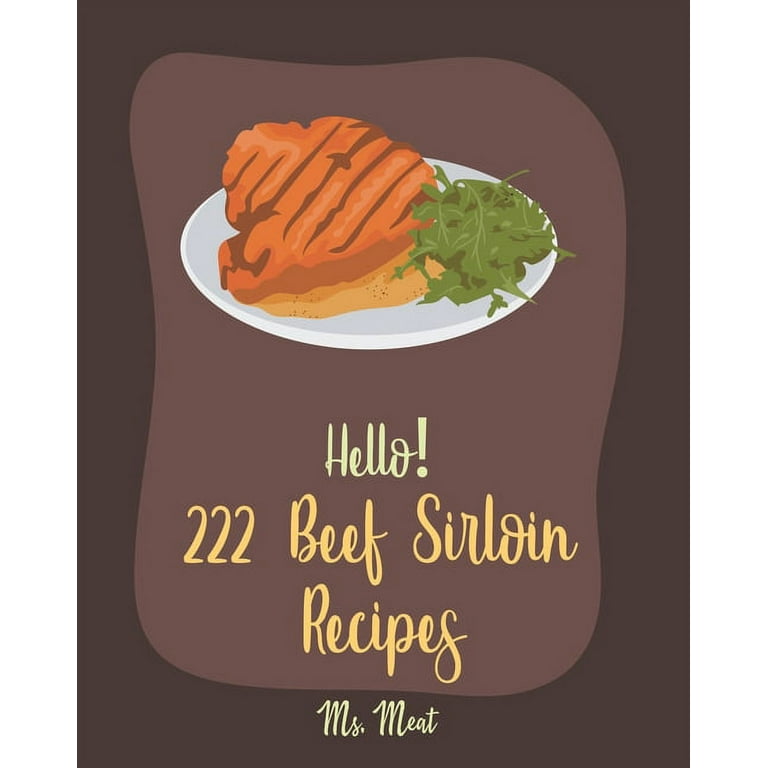This computer-generated advertisement features a central white plate of food against a backdrop of dual purple shades, with the inner shade being a lighter purplish-brown and the outer one almost black. On the plate is a char-grilled piece of beef sirloin, placed atop an orange substance that might be a gravy, accompanied by a pile of green leafy vegetables. The cursive text on the image reads, "Hello!" in bright yellow, followed by "222 Beef Sirloin Recipes" in a deeper yellow, and then "Miss Meat" in the same bright yellow color, enhancing the visual appeal of the overall design.